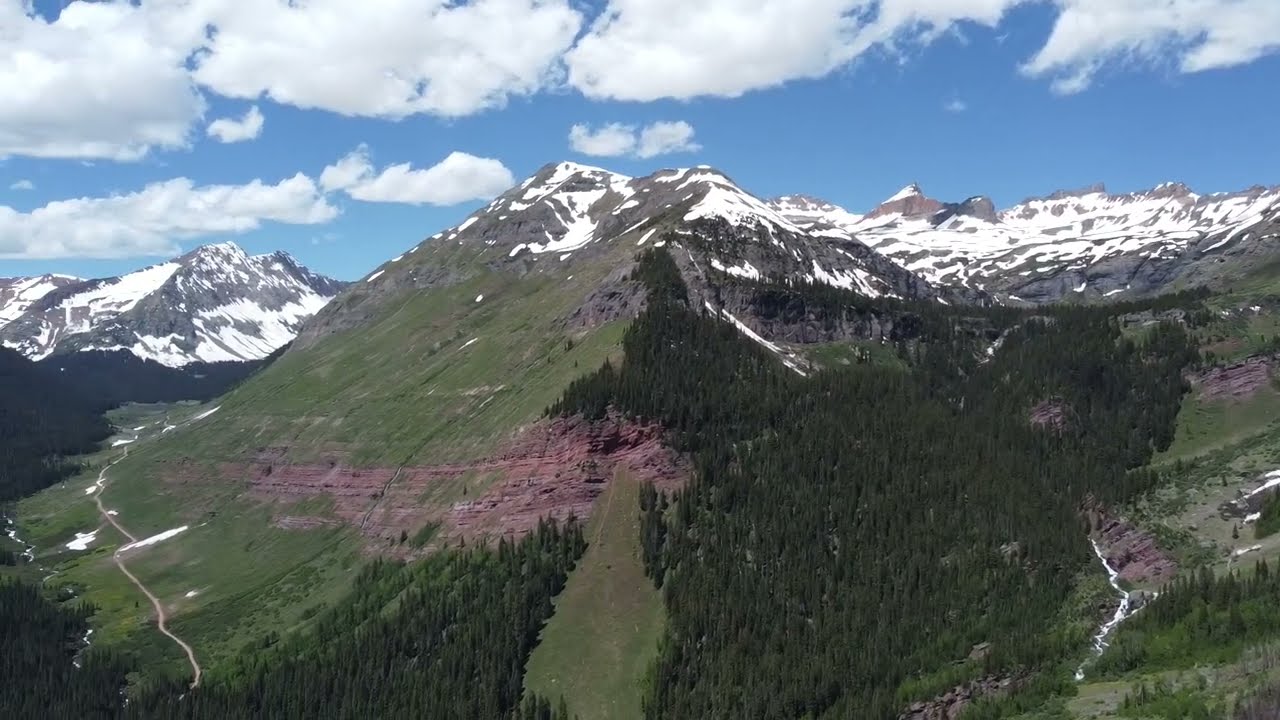The photograph captures a breathtaking view of a snow-capped mountain range on a partly cloudy day. The image is horizontally aligned and portrays a vivid blue sky adorned with puffy cumulus clouds. Dominating the center of the image is a prominent grayish-brown mountain peak, its summit dusted with snow. To the left, the mountainside reveals a smooth grassy area interspersed with patches of white snow. In the distance, shorter mountain peaks echo the snow-covered motif.

The terrain at the bottom of the photograph features tall green pine trees densely lining the lower portion and extending towards the right side of the image. A winding road, resembling a squiggly line, snakes through the forested areas, visible both at the bottom and to the right of the main peak. Adding to the intricate landscape, a scar of terraced red dirt disrupts the greenery towards the lower middle left of the image. 

Overall, the photograph encapsulates the raw beauty of the mountainous landscape with a harmonious blend of dark green, brown, gray, white, and light blue hues, emphasizing the serene and majestic outdoor setting.